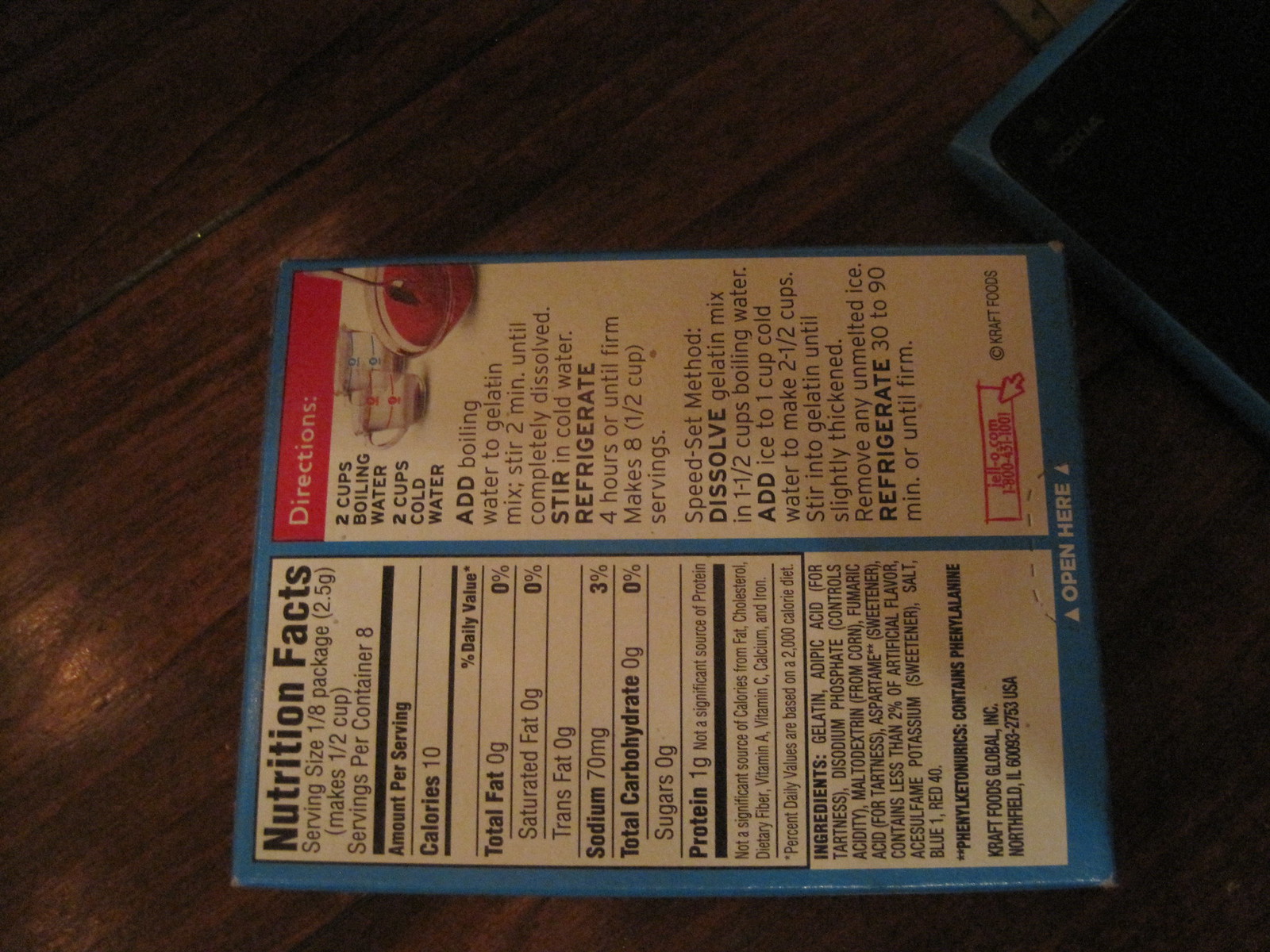The image depicts a color photograph of a product label, specifically the back label of what appears to be a Jell-O package, placed on a brown wooden table. This label, seemingly cut out from the original packaging and turned to its side, features a blue edge. The left side of the label displays nutritional facts, including specifics such as eight servings per container, each serving making half a cup, containing 10 calories, 70 milligrams of sodium, and no carbohydrates or sugars. The first ingredient listed is gelatin, confirming the product is Jell-O. The right side showcases the preparation directions, detailing the use of two cups of boiling water followed by two cups of cold water. There is also a small, somewhat unreadable panel at the bottom instructing "Open Here". Additionally, there's an image at the bottom right corner of the label showing Jell-O in a clear bowl with a spoon on top. The scene includes a partial view of a cell phone with "Nokia" inscribed, adding context to the tabletop setting.